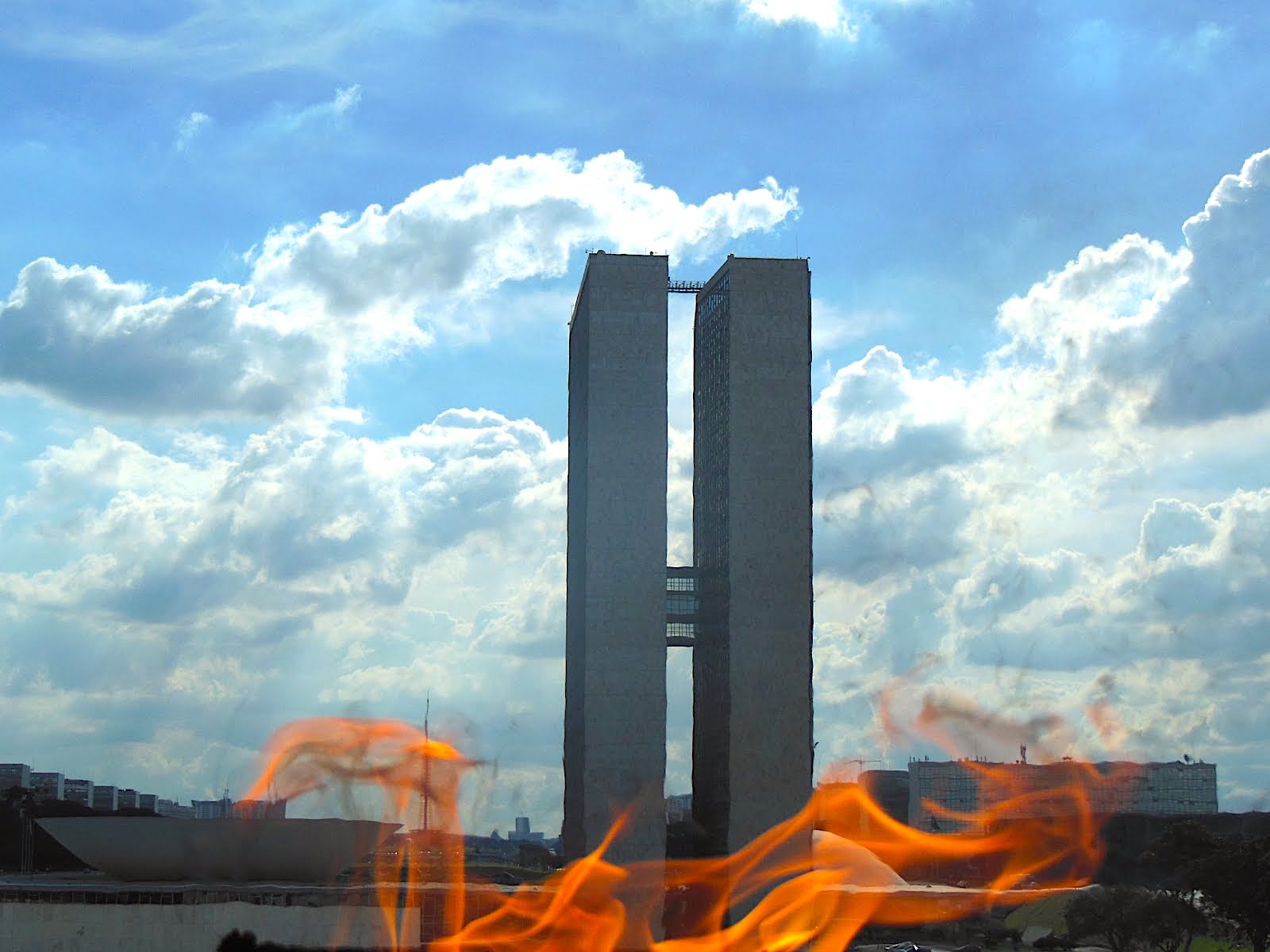In the center of this landscape-oriented color photograph, two large, identical, dark gray buildings dominate the scene. The architectural structures are connected by a passageway situated midway up and a smaller walkover near their tops, suggesting potential pedestrian access between the towers. The sky, a vibrant blue adorned with numerous puffy white clouds, occupies most of the background, enhancing the verticality of the buildings. Below, the foreground features a vivid orange flame, slightly obscuring the base of the towers and adding a dramatic element to the image. Additional smaller buildings and structures, including what may be a docked boat, populate the lower section of the photograph. The overall setting appears to be a mix of commercial and residential areas, captured with photographic realism. No text is present in the image, and the color palette includes shades of blue, white, gray, orange, yellow, and black.